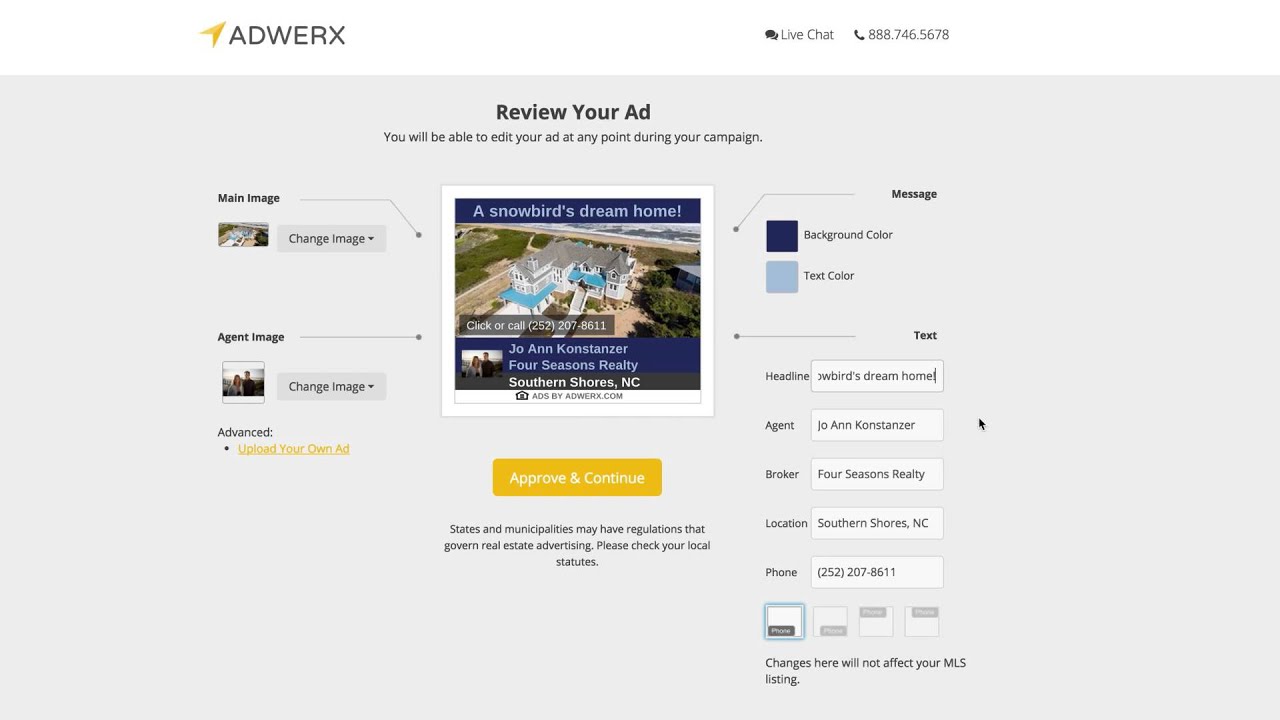**ADWERK Website Interface for Ad Review and Editing**

The ADWERK homepage prominently features a comprehensive ad review and editing interface. In the upper right corner, visitors are provided with a "Live Chat" option and a customer service number (888-746-5678) for immediate assistance. 

Centrally located on the site is a clear directive: "Review Your Ad." This section allows users to edit their advertisements at any point during their campaign. Users can interact with various ad elements, predominantly found on the left side. Here, you'll find options labeled "Main Image" and "Agent Image," each accompanied by a dropdown menu that lets users change these images as needed.

On the left-hand side, users can visualize the images linked to their ad, while an "Advanced" section provides further customization options, such as adding bullet points or uploading their own ads. The link "Upload Your Own Ad" is highlighted in yellow and underlined for easy identification.

The central part of the interface displays a sample advertisement with a picturesque image labeled "Snowbird's Dream Home." It encourages viewers to click or call 252-207-8611 to contact Joanne Cozzaner from Four Seasons Realty, located in Southern Shores, North Carolina. The image also features a small attribution to adsbyadwerk.com.

At the bottom center of the interface, a yellow button labeled "Approve and Continue" invites users to finalize their ad. A note below this button advises users to check their local statutes, as regulations that govern real estate advertising may vary by state and municipality.

On the right side of the interface, there's a section illustrating ad message specifics, displayed in varying shades of blue. This includes text elements like "Text" and "Headline," with the sample headline reading "Snowbird's Dream Home" in distinct light blue text.